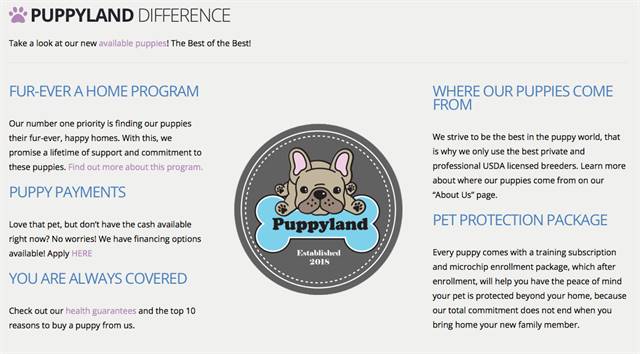The image features a background entirely shaded in a tannish beige color. In the upper left corner, there is a prominent purple paw print accompanied by the text "Puppy Land Difference" written next to it. Below this, in smaller font, the phrase "Take a look at our new available puppies, the best of the best" is displayed. Directly underneath, in bold blue capital letters, it reads "Forever a Home Program." Additional text mentions "puppy payments" and reassures that "you are always covered."

On the right side of the image, the phrases "Where our puppies come from" and "Pet Protection Package" are clearly visible. 

At the center of the image, a logo stands out—a dark gray circle with a white border circle inside it, followed by a dotted circle. Within these circles, an illustration of a dog, resembling either a pug or a French Bulldog, is depicted. The dog, which has a tannish coat, brown nose, and pink inner ears, is shown lying on its stomach and looking forward.

Below this logo, there is a blue dog bone graphic with the text "Puppy Land" inscribed on it in white font. Beneath "Puppy Land," the establishment year "Established 2018" is written, completing the image's detailed elements.